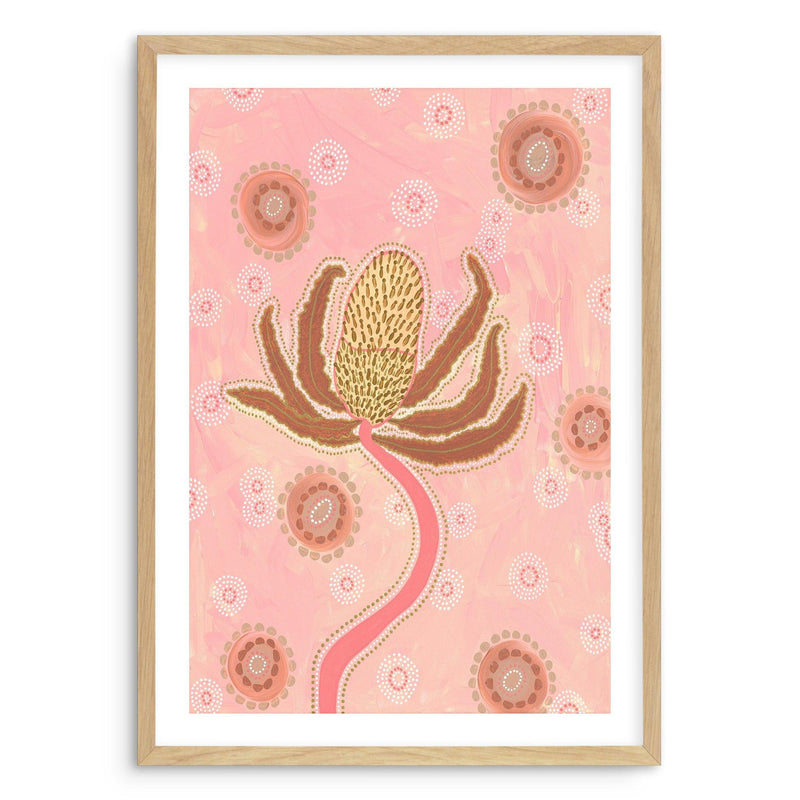This portrait-oriented painting showcases a flower with a pink stem and green leaves, framed by a light brown wooden frame with a white inner border. The flower's central bulb features vibrant yellow and pink hues, surrounded by thin, elongated, feather-like petals. The background is predominantly pink, subtly accented with watercolor-like touches of yellow. Floating around the stem and flower are numerous circular patterns: around 20 white circles with pink centers organized from the bottom to the top, and six larger pink circles that have darker pink dots in their centers and are encircled with green dots. These elements create a whimsical, dandelion seed effect, contributing to the artwork’s intricate and delicate aesthetic.